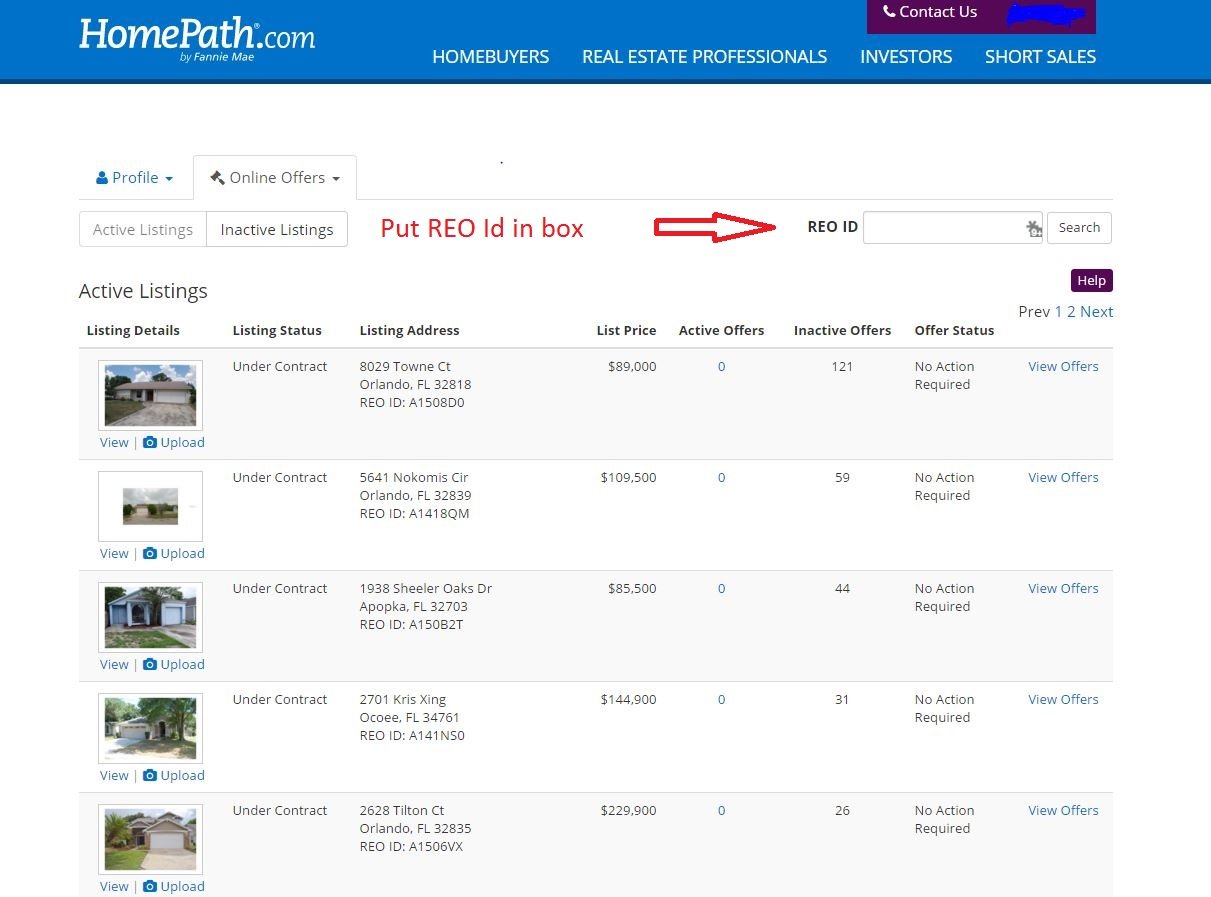This detailed description captures the entirety of the webpage from HomePad.com. The landing page features a prominent blue rectangular bar at the top, which includes the website's name and the main menu. The menu options listed are: Home Buyers, Real Estate Professionals, Investors, and Short Sales, with an additional link to contact the team.

Beneath the main menu lies another section with smaller navigation links: Profile, Online Office, Active Listing, and Inactive Listing. Adjacent to this, there is a search box for entering an REO ID, clearly indicated by a red arrow.

The core content of the page consists of property listings. Each of the five displayed homes includes a thumbnail image and essential information on a single row. This includes the property's status, address, price, and office status (active or inactive). Pagination options are provided at the bottom with labels for previous, page 1, page 2, and next, helping users navigate through multiple listings.

The text accompanying the images of the homes is written in light blue, while the remainder of the informational text is in black, ensuring clear readability and distinction.